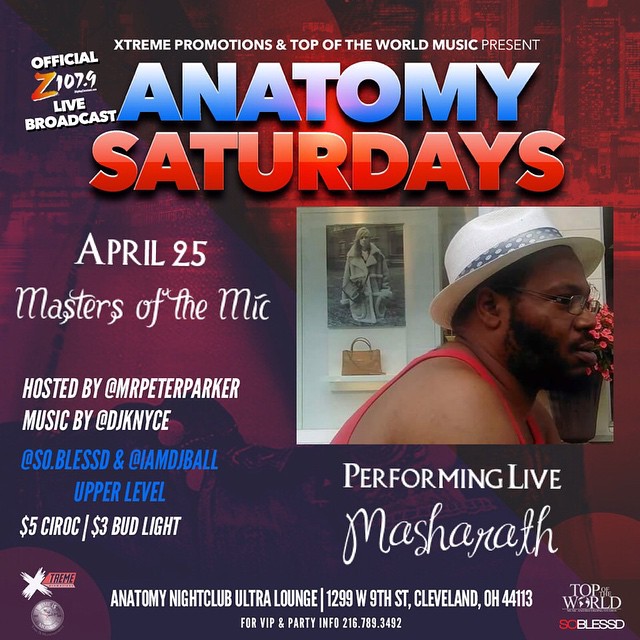This image is a detailed flyer promoting "Anatomy Saturdays," an event featuring a live broadcast by Official Z107.9. The banner, adorned with blue and red 3D effect letters, prominently displays "Anatomy" in blue and "Saturdays" in red. Above the title, in white font, reads "Extreme Promotions and Top of the World Music Present." The left side of the flyer announces "April 25th, Masters of the Mic," and highlights that the event is hosted by Mr. Peter Parker with music by DJ KNYCE. 

A pivotal visual element of the flyer is the image of a man wearing a red tank top and a white fedora with a black brim, positioned on the right. Behind him, a somewhat golden picture of a lady in a fur coat holding a purse adds to the graphical appeal. Additional text in various blue letters includes promotional handles like "soblessd" and "iamdjballupperlevel."

The flyer also mentions some practical details: it costs $5 to attend and Bud Light is priced at $3. It specifies the nightclub location and includes logos from various sponsors, ensuring a comprehensive promotional display.